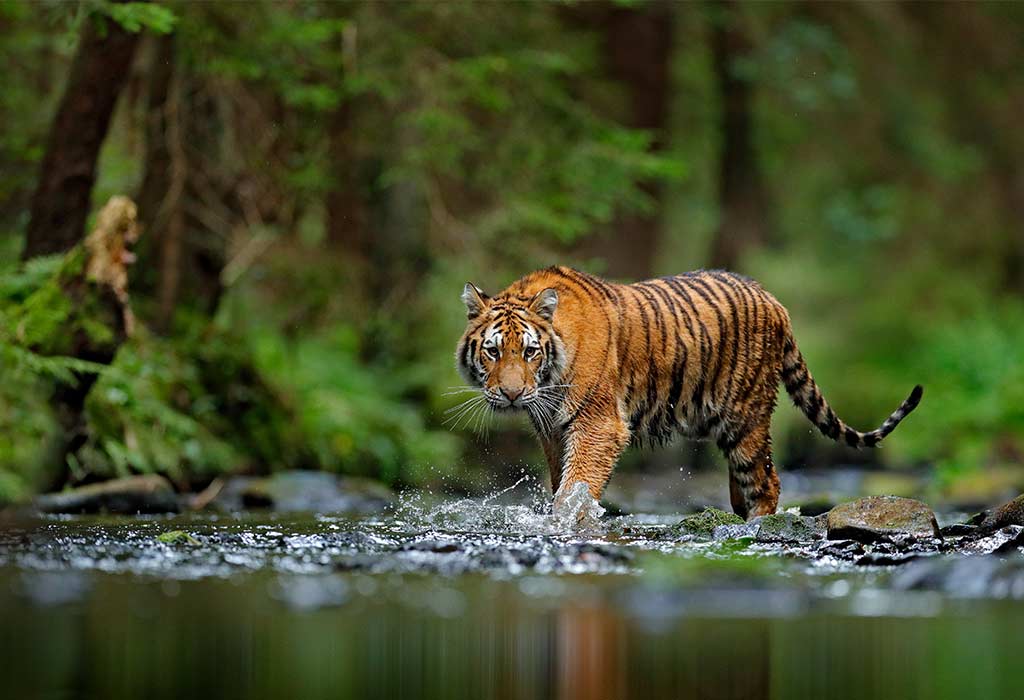This outdoor photograph captures a majestic tiger walking through a shallow creek in a dense jungle setting. The tiger, with its vibrant orange fur and striking black stripes, is prominently featured as it moves through the water, creating a dynamic splash with its front left paw. The water droplets can be seen clinging to its lower body, tail, and belly, indicating it has been wading through the creek for some time. The tiger's powerful build is highlighted, showcasing its defined muscles and distinct whiskers as it gazes forward, seemingly aware of the camera. Surrounding the tiger is a lush backdrop of greenery, including low trees, bushes, and various plants. The background is slightly blurred, drawing more focus on the tiger but still displaying the trunks and bark of the forest trees. On the creek bank, partially submerged jagged rocks add texture to the scene, enhancing the wild and rugged environment of this jungle habitat.